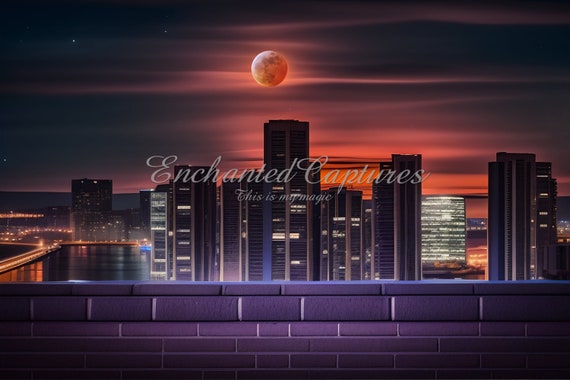The image is a stunning digital render or piece of digital art depicting a nighttime cityscape from the top of a high-rise building, possibly around 30 to 40 stories high. In the foreground, a brick wall or barrier suggests the vantage point, while the background reveals a sea of illuminated tall buildings, their windows alight, piercing the night. Hovering above this urban expanse is a mesmerizing reddish-colored moon, casting a radiant red glow that spans across the skyline, subtly bathing the city below. To the left of the image, a small bay reflects the dazzling lights from above, intersected by a street or bridge crossing through the water. The sky enhances the magical atmosphere with a sprinkling of tiny white stars around the glowing moon. The overall scene is not just a visual feast but an 'enchanted capture,' as indicated by the words etched on the image, suggesting the photographer-artist's intent to evoke the sense of magic in a moonrise over a bustling city.